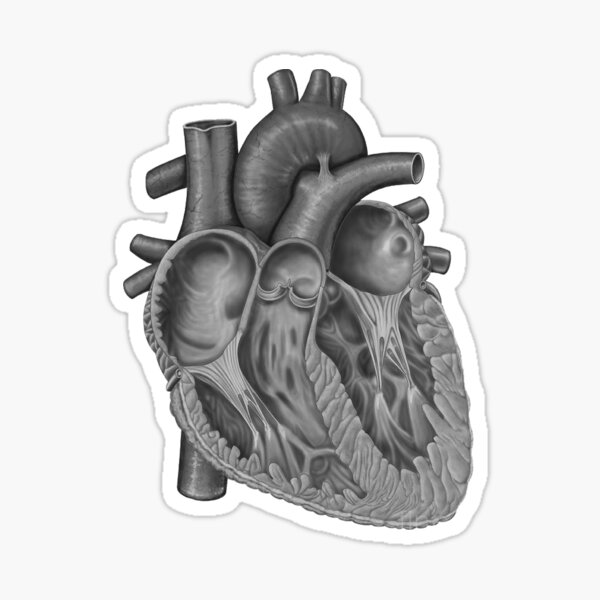The image represents an artist's detailed anatomical illustration of a bisected human heart, framed as though it were a sticker. It features a cross-section of the organ, rendered in varying shades of gray to highlight its intricate internal structures. The heart is centrally positioned against a very light grey background and is bordered by a thin white band, accentuating its edges. The drawing meticulously showcases the muscle walls, different chambers, ventricles, and the open-ended arteries and veins that terminate abruptly, indicative of the segmentation from the rest of the cardiovascular system. The valves and the major arteries such as the aorta are discernible, enhancing the diagrammatic quality of this art piece that could easily pass as a detailed textbook illustration. Its grayscale palette and precise detailing, along with the white outline, give it the appearance of a sticker, making the heart appear almost as though it is floating against the pale backdrop.